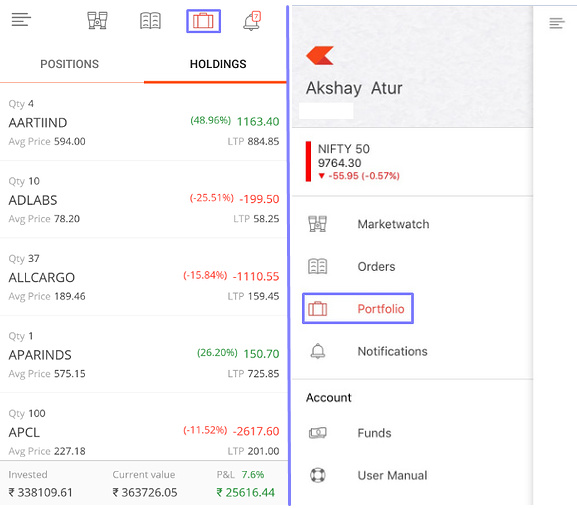Here's a detailed and cleaned-up caption for the given content:

---

The image displays a portfolio summary with detailed stock holdings and their respective performance metrics:

1. **AARTIND**:
   - **Positions**: Holdings
   - **Quantity**: 48.96%
   - **Average Price**: $594.00
   - **Total Investment**: $1,163.40
   - **Last Traded Price (LTP)**: $884.85

2. **ADLabs**:
   - **Quantity**: 10 shares
   - **Average Price**: $78.20
   - **Performance**: -25.51%
   - **Unrealized Loss**: -$199.50
   - **LTP**: $58.25

3. **AllCargo**:
   - **Quantity**: 37 shares
   - **Average Price**: $189.46
   - **Performance**: -15.84%
   - **Unrealized Loss**: -$1,110.55
   - **LTP**: $159.45

4. **APA Holdings**:
   - **Average Price**: $575.15
   - **Performance**: +26.20%
   - **Unrealized Gain**: $150.70
   - **LTP**: $725.85

---

This detailed caption provides a clear and comprehensive view of the investment portfolio's current status.